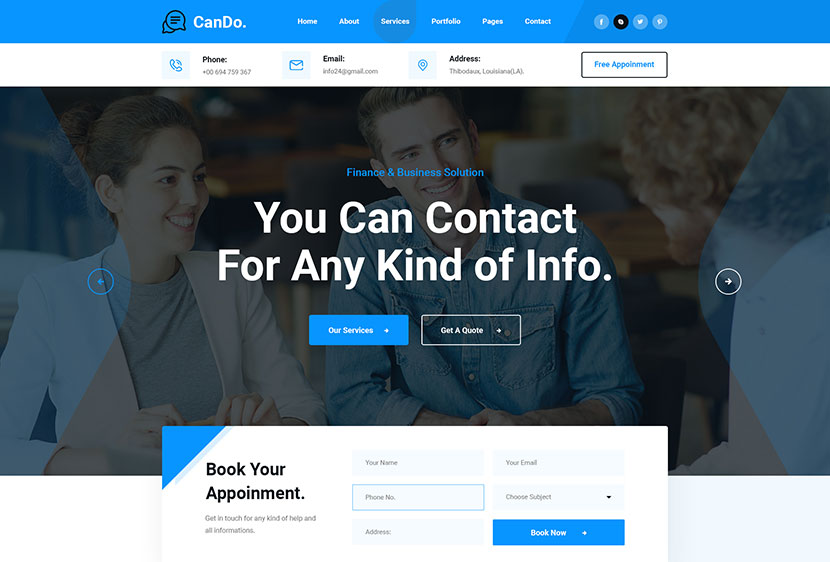The image showcases a website called "CanDo," with the name displayed in white text on a blue navigation bar at the top, spanning from left to right. The navigation bar includes several options: "Home," "About," "Services," "Portfolio," and "Contact." The "Services" option is highlighted within a dark blue circle.

Social media icons for Facebook, Twitter, and two others, including one in black, are displayed prominently on the site. Contact information, including the phone number, email address, and physical address, is provided below these icons. A black box with white text features the phrase "Free Appointment" in blue.

The main section of the website features an image of a smiling woman and man, sitting next to each other and seemingly engaged in conversation, possibly with another person. Accompanying the image is text stating, "Contact for any kind of info," along with "Finance and Business Solution." 

Below the image, there are two call-to-action buttons: a blue one labeled "Our Services" and a clear one labeled "Get a Quote." Further down, a white box with a blue triangle in the upper left corner reads "Book Your Appointment." Smaller text advises visitors to get in touch for help and information.

The site includes fields for visitors to enter their name, phone number, address, email, and subject choice. Below these fields, in a blue box, is another call-to-action button labeled "Book Now."